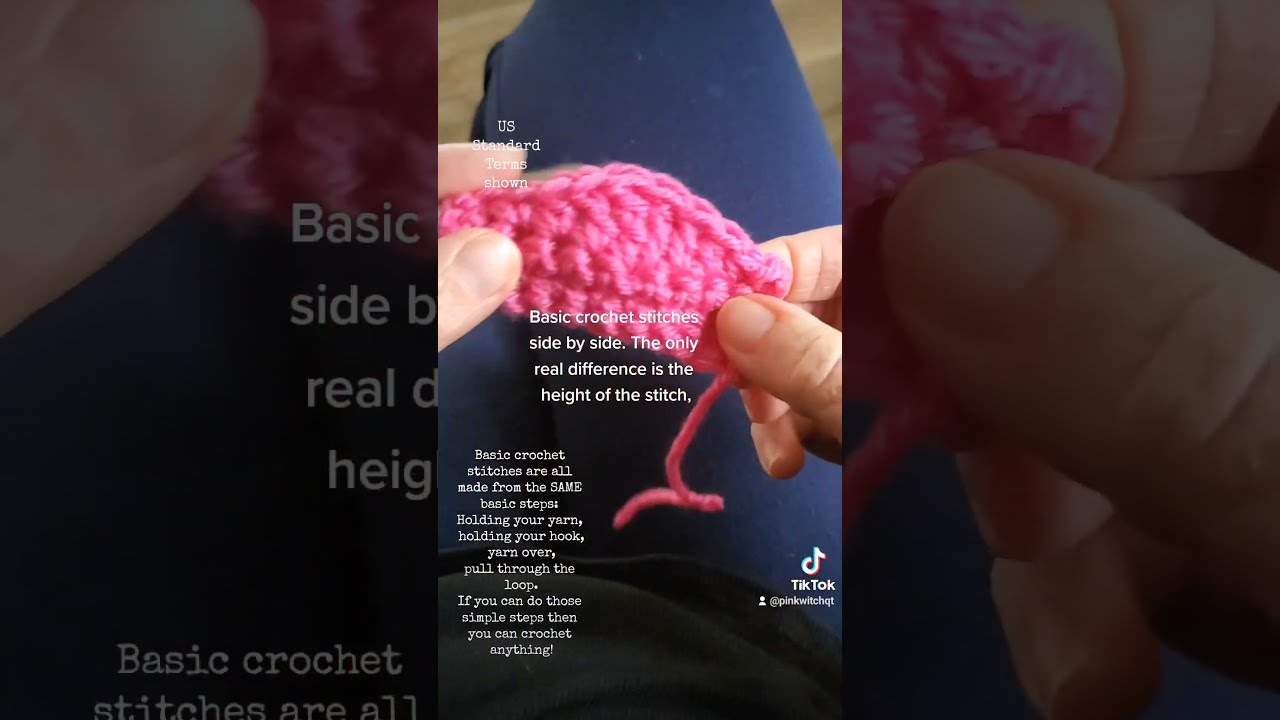In this screenshot taken from a TikTok video, we see a detailed tutorial on basic crochet stitches. The video features a person's hands working on a small piece of pink crocheted fabric, demonstrating the basic techniques of crocheting. The individual is wearing blue pants and sitting cross-legged on wooden floors, with their hands prominently featured as they hold the crochet hook and yarn. Several captions in white text are overlaid on the image, explaining the process: "US standard terms shown. Basic crochet stitches side-by-side. The only real difference is the height of the stitch. Basic crochet stitches are all made from the same basic steps: holding your yarn, holding your hook, yarn over, pull through the loop. If you can do those simple steps, then you can crochet anything." The TikTok logo and handle (@pinkwitchitQT) are visible in the bottom right, indicating this is from a crafty TikTok channel. The screenshot also shows the same video enlarged and darkened behind the main image to provide additional focus on the instructional content.